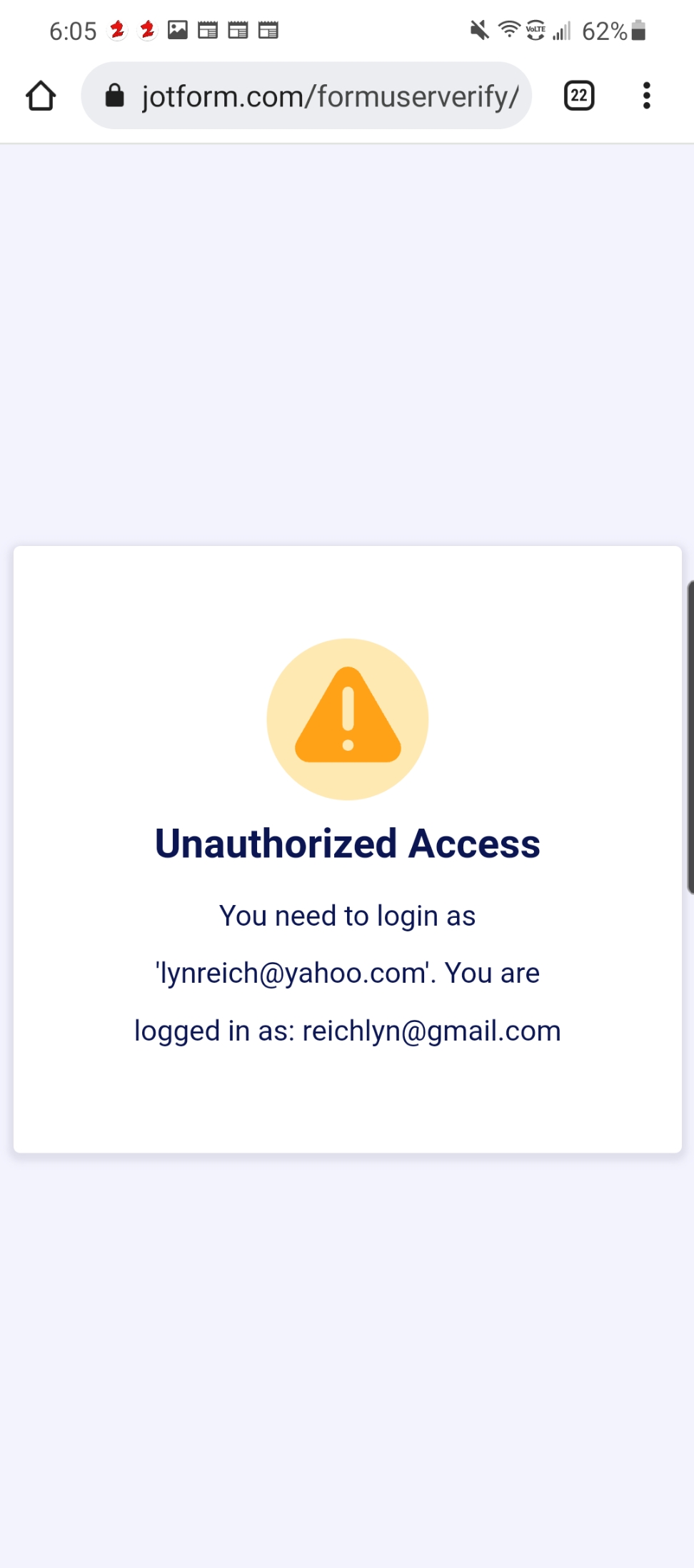This image appears to be a screenshot taken from a cell phone. The overall background of the screen is a deep, purplish-blue color, skewing more towards purple. Centrally positioned is a white, rectangular pop-up message.

At the top of this message is a yellow exclamation point encased in an orange triangle, which itself is circled in yellow. The bold black text within the message reads: "Unauthorized Access." Below this, in standard black font, the message continues: "You need to log in as lynnreich@yahoo.com. You are logged in as reichlynn@gmail.com." The text "lynnreich@yahoo.com" is enclosed in quotation marks for emphasis.

For context, at the very top of the screen outside the message box, the web address being visited is visible as "jotform.com/formuserverify/". In the status bar, the time displayed is 6:05 and the battery level indicates 62% remaining.